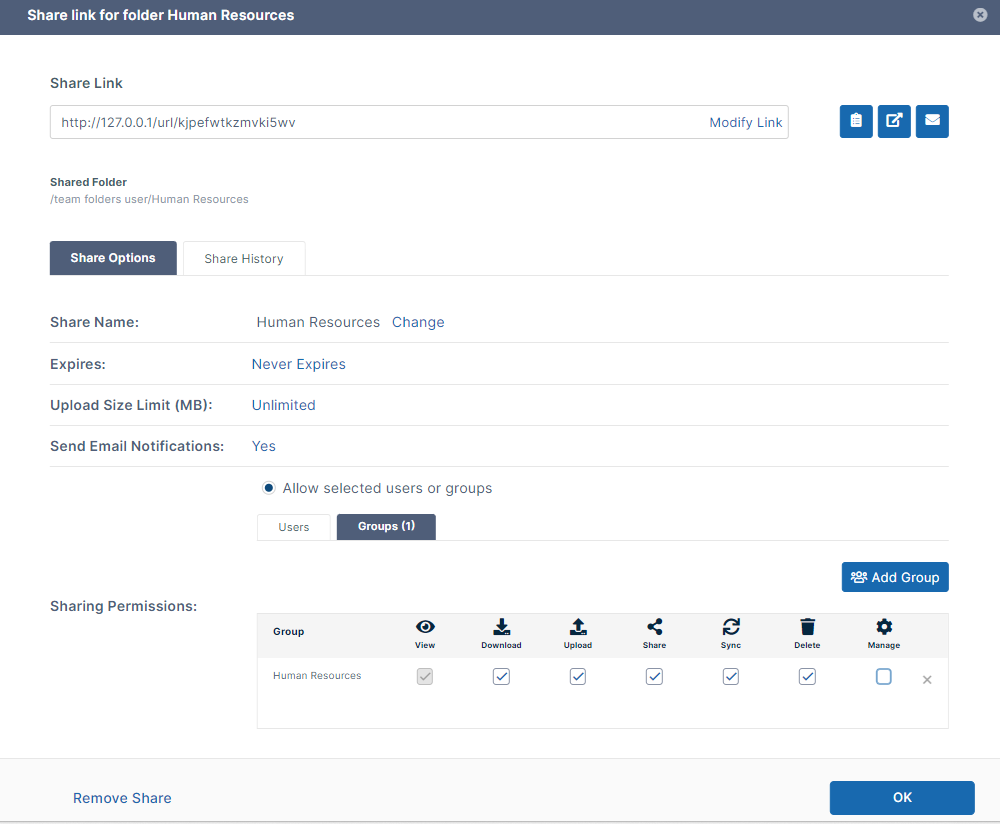The image depicts a file-sharing interface for a "Human Resources" folder. At the top, there is a dark blue rectangle banner that spans the width of the screen, featuring the text "Shared Link for Folder: Human Resources" in white, with a small 'X' button situated in the top right corner. 

Below the banner, there is a section with "Shared Link" in black text and a bar for adding a link, accompanied by three blue squares to its right. Further down, captions read "Shared Folder," followed by options labeled "Share Options" and "Share History."

On the left side of the interface, there is black text listing various details: "Share Name," "Expires," "Upload Size Limit (MB)," and "Send Email Notifications." Adjacent to this, in gray text under "Human Resources," are the statuses "Change," "Never Expires," "Unlimited," and "Yes." 

Below, there is a prompt to "Allow Selected Users or Groups," with "Users" and "Groups" tabs to the right, the latter being highlighted, showing the number one.

At the bottom of the panel, there are seven icons indicating sharing permissions: "View," "Download," "Upload," "Share," "Sync," "Delete," and "Manage." Each is highlighted in black, with six of them checked off, except for the last icon on the right.

Towards the bottom left corner, there is an option to "Remove Share" in blue text. In the bottom right corner, there is an "OK" button in white text against a blue background.